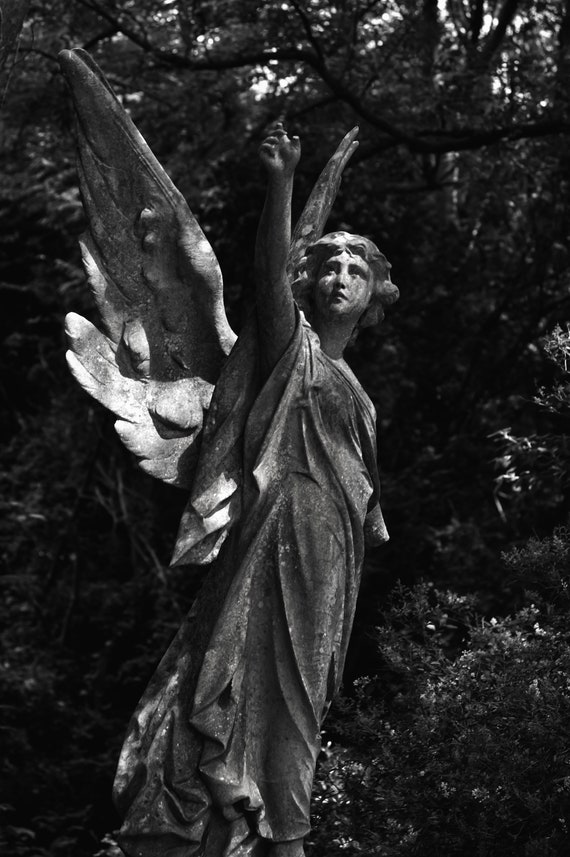In this black-and-white photograph, we see a meticulously carved marble statue of an angel, positioned outdoors against a backdrop of dense, shadowy trees and shrubbery, identifiable by the intricate leaf patterns and texture. The angel, whose gender is indeterminate, has a body that faces the right side of the image, while the head is turned upwards, offering a full view of its weathered face. The angel’s right arm is extended skyward, with the eyes following the hand’s reach, although several fingers have been broken off, indicating age and damage. The statue’s large wings spread diagonally across its back, enhancing the angelic depiction. The figure is adorned in a flowing, intricately detailed robe, with visible ripples and creases in the fabric, and the right arm protruding from the garment. The overall scene captures a moment of celestial aspiration, marred slightly by time's erosive touch.